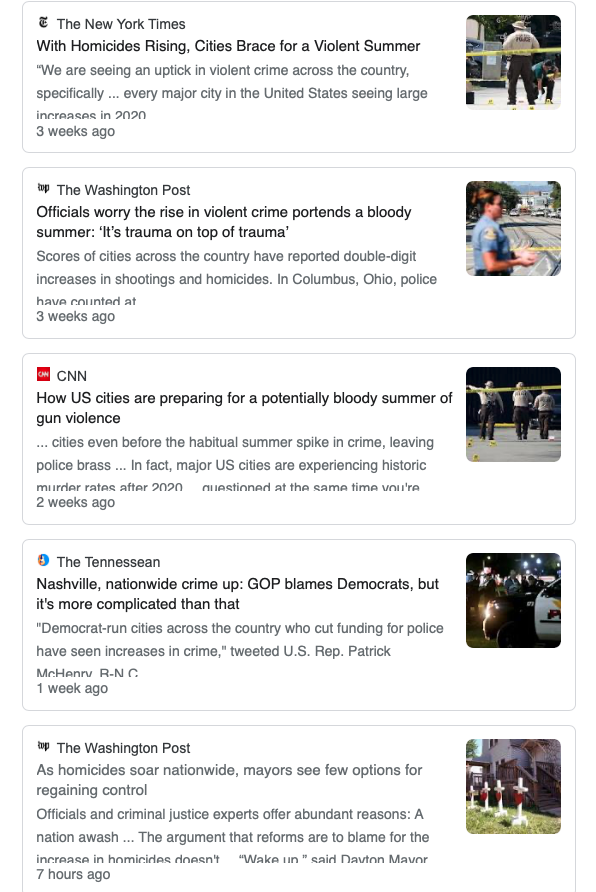Here is the updated and detailed caption for the image:

---

"This image captures a typical online news feed as seen on platforms like Google News or the Bing homepage. The page features five articles from prominent news organizations, addressing the rising issue of violent crime in U.S. cities.

1. **New York Times**: The headline reads, *'With homicides rising, cities brace for a violent summer.'*
2. **Washington Post**: The next headline follows a similar theme with, *'Officials worry the rise in violent crime portends a bloody summer.'* 
3. **CNN**: Another article echoes these concerns, emphasizing a *'trauma on top of trauma.'*
4. **The Tennessean**: Continuing the narrative of increasing violence, this news piece also refers to a *'bloody summer.'*
5. **Washington Post again**: The second article from the Washington Post reiterates the same alarming prediction of a *'bloody summer.'*

As observed, multiple articles use the term 'bloody summer', suggesting a coordinated emphasis on the anticipated increase in violent crime during the summer. This convergence of messaging points to potential shared talking points across different news outlets."

---

This caption provides a comprehensive and clear description, suitable for a reader who is not viewing the image.